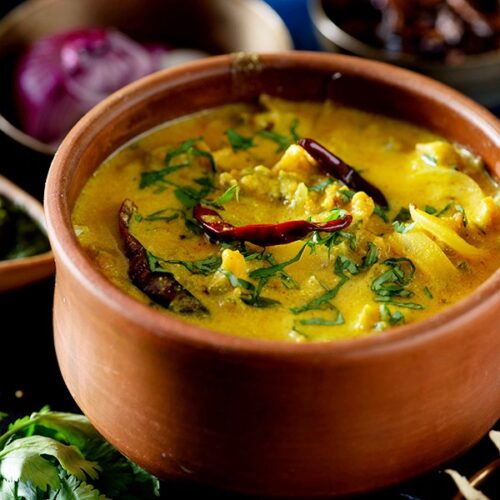This close-up photograph, suitable for a food-focused cookbook or magazine, showcases a vibrant, thick soup served in a brown terracotta bowl. The bowl, roughly eight inches in diameter, cradles a robust yellow broth reminiscent of a curry or flavorful gumbo. Garnishing the top of the soup are finely chopped onions and vivid burgundy chili peppers, adding a touch of heat and color contrast. Fresh green herbs, possibly cilantro or parsley, are sprinkled delicately, enhancing the visual and aromatic appeal. In the slightly blurred background, an array of ingredients and kitchenware, including a leafy vegetable underneath the bowl and a whole red onion awaiting preparation, set a warm and inviting culinary scene.